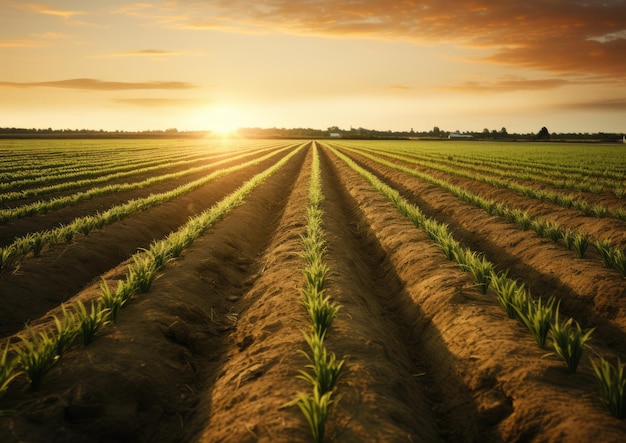This vividly detailed image showcases a meticulously depicted farm field, possibly a photograph or digital rendering, laid out in a landscape format. The scene is oriented with rows of green plants, likely some form of crops or grass, planted in elongated mounds of brown dirt, each mound approximately a foot apart. These rows extend symmetrically towards a vanishing point on the horizon, creating a sense of depth and continuity across the image. The troughs between the mounds create a series of shadows, accentuating the ridged texture of the field.

In the top third of the image, the sky transitions from a light blue on the left to a sunlit, bluish-orange hue, indicating either sunrise or sunset. Rich clouds, darker on the right, are illuminated from below, adding to the dramatic atmosphere. Just left of center on the horizon, a bright sun is partially visible, casting a warm glow over the landscape. Below the sun, a thin, distant line of low hills dotted with trees and sporadic buildings can be seen, providing a backdrop to the expansive farmland. Together, these elements create a harmonious blend of natural and possibly artificial beauty, reflecting a tranquil yet dynamic rural setting.